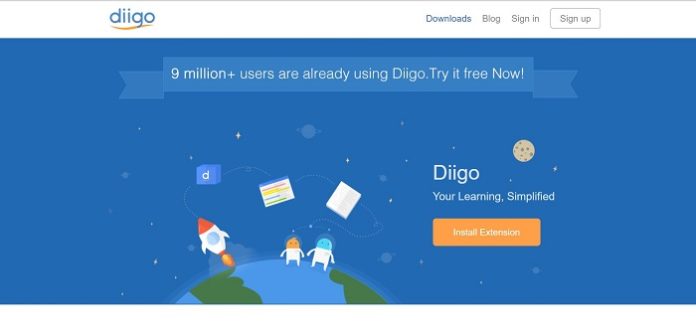The webpage for Diigo, featuring a bold and vibrant design, presents a striking visual to its 9 million+ users. Dominating the page is a blue-colored, computer graphic-style poster, which serves as the background. This scene includes two whimsical, cartoonish aliens standing on a miniaturized Earth. Adjacent to them stands a rocket, suggesting an interstellar voyage. Above the Earth, stars twinkle subtly throughout the sky. 

At the top, a white navigation bar provides links for 'Downloads,' 'Blog,' 'Sign In,' and 'Sign Up.' An orange button inviting users to "Install Extension" adds a touch of contrasting color. Adding to the celestial backdrop, a moon resembling a chocolate chip cookie appears in the distance, along with several planet-like graphics, including multiple renditions of Saturn with its iconic rings.

This playful and engaging illustration emphasizes the platform's tagline: "Diigo, Your Learning Simplified," encouraging users to explore the free service.